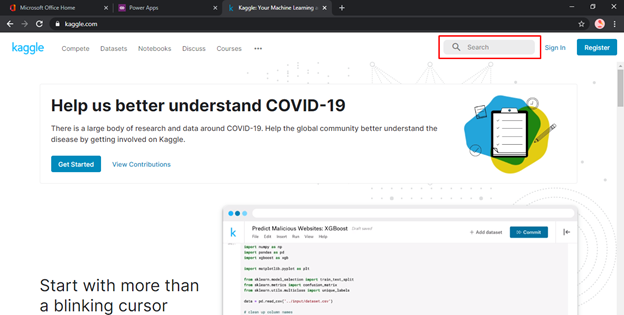A web browser window with multiple tabs open is displayed, showcasing an active session on Kaggle.com. The tabs include Microsoft Office Home, Power Apps, and Kaggle, a platform for data science and machine learning. The Kaggle webpage that is currently open highlights several features and sections. 

In the top right corner of the Kaggle page, a search button is outlined in red, indicating a focus on its usability for training purposes. Beside the search button are two blue buttons: one for "Sign In" and another labeled "Register," both with clean white text. The Kaggle logo, with its distinctive blue lettering, is also situated in the upper right-hand corner.

The navigation menu spans from left to right, featuring the options "Compete," "Datasets," "Notebooks," "Discuss," "Courses," and a three-dot context menu for additional settings. Below this menu, a prominent announcement is displayed, urging users to help better understand COVID-19, accompanied by clipboard-themed artwork on the right-hand side. The message encourages the global community to contribute to research around COVID-19, with a "Get Started" button in a blue box with white text conveniently placed for easy access.

Further down, a section titled "Start with more than a blinking cursor" is visible, suggesting the availability of resources to aid new users in coding. An example coding page is also shown, reinforcing Kaggle's role as a supportive platform for coding and data science endeavors.